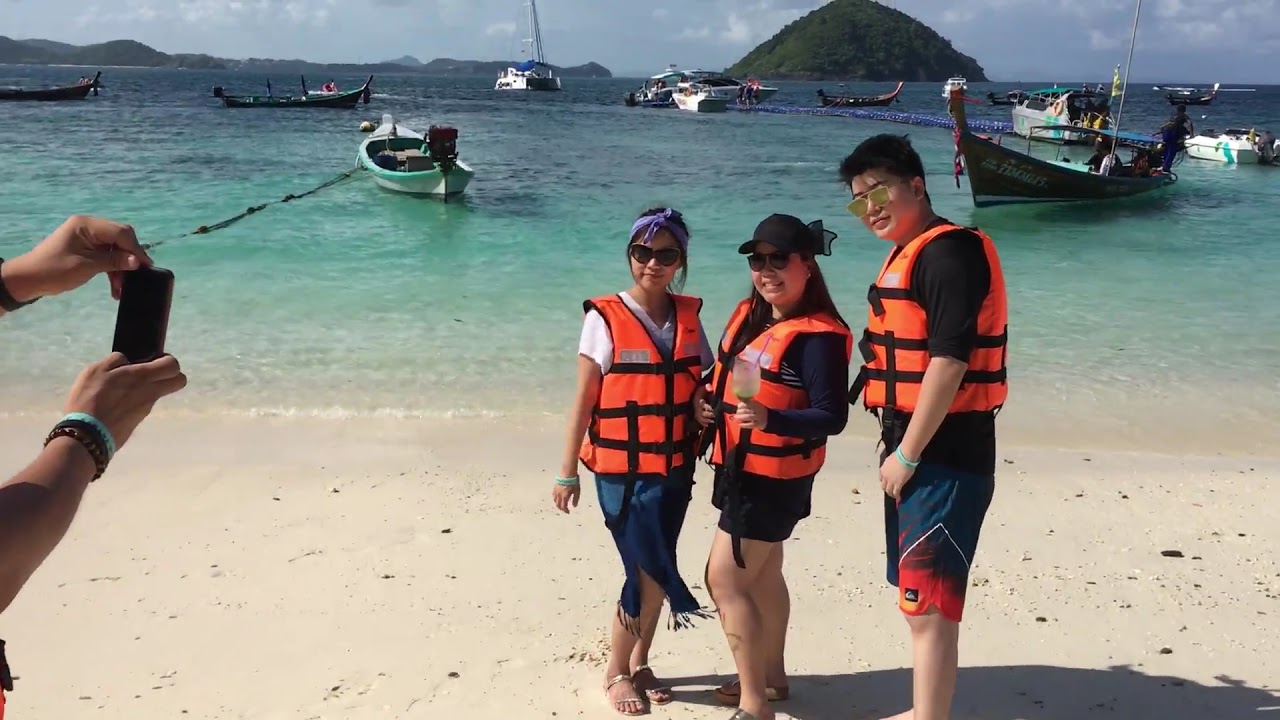In this horizontally aligned rectangular image, three young Asian friends are posed for a photo on a light tan sandy beach. They are all wearing orange life vests with black bands. The man on the right has short black hair and is sporting yellow sunglasses, a short-sleeve black shirt, and blue and red swim trunks. The woman in the middle wears a black baseball cap, black sunglasses, a black top, and orange shorts while holding a drink in her left hand. The woman on the left has black hair pulled back with a purple tie around her head, black sunglasses, a short-sleeve white shirt, and a blue skirt with tassels, along with sandals. 

In the background, a large body of clear blue water gradually deepens from light blue to dark blue, dotted with at least thirteen boats, mostly canoes and small fishing vessels. On the left side of the image, you can see a pair of hands, wearing bracelets, holding a phone to take a photo of the three friends. Further back, there are tall grassy hills in the middle of the ocean, land outlines, and a blue sky with some white clouds. A slightly larger brown boat with a white line on the bottom sits closer to the shoreline, with two people inside, and more boats are visible further out in the water. This serene outdoor beach setting captures a moment of friendship and adventure.